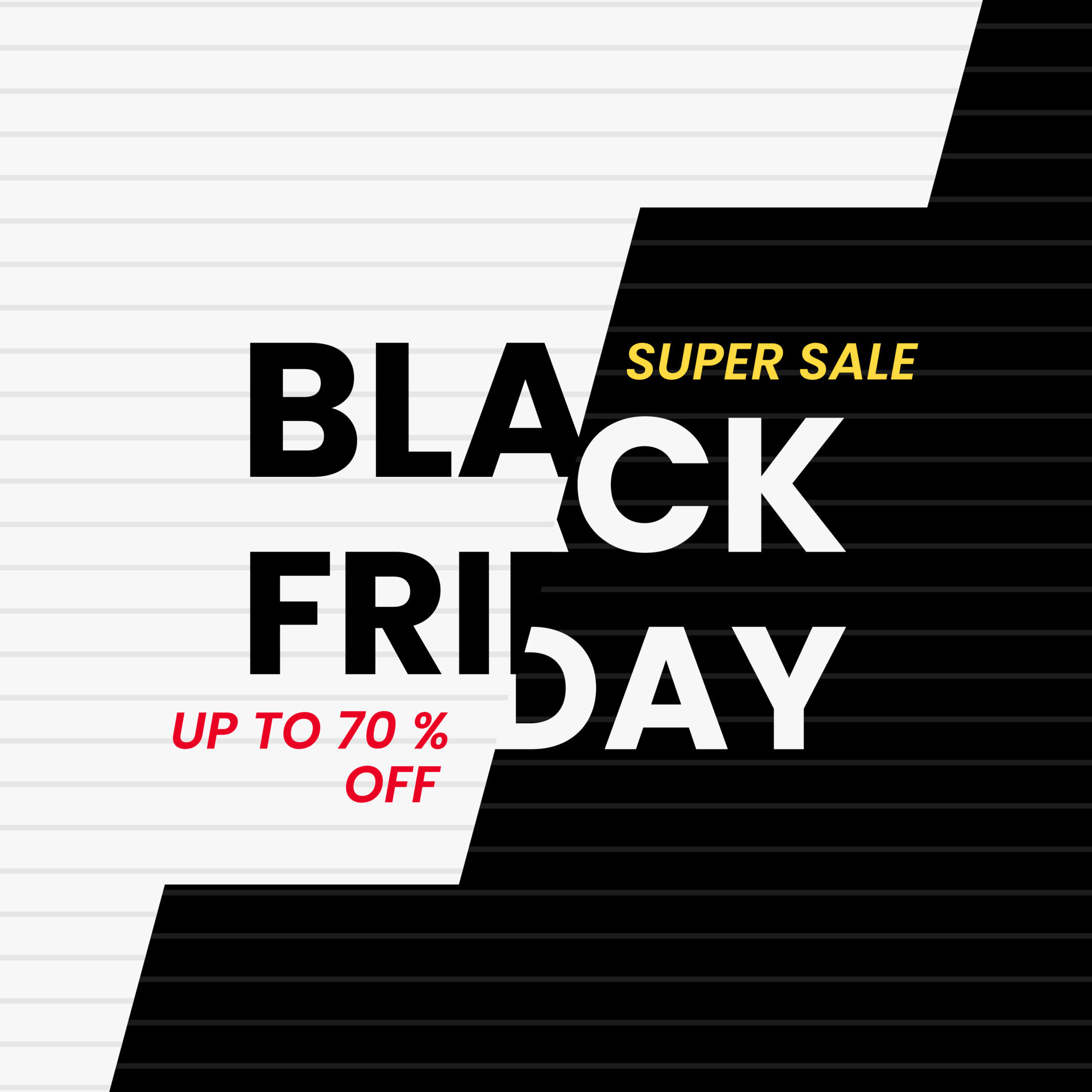This image advertises a Black Friday super sale with bold and striking text. The background is split diagonally, with the top left half in white featuring horizontal gray lines, and the bottom right half in black. Dominating the center, the phrase "Super Sale" is prominently displayed in yellow letters. The text "Black Friday" is split with "BLA" in black and "CK" in white, "FRI" in black, and "DAY" in white. Additionally, the offer "Up to 70% Off" is highlighted in vibrant red letters beneath the "FRI." The layout and color scheme effectively draw attention to the major sale event.